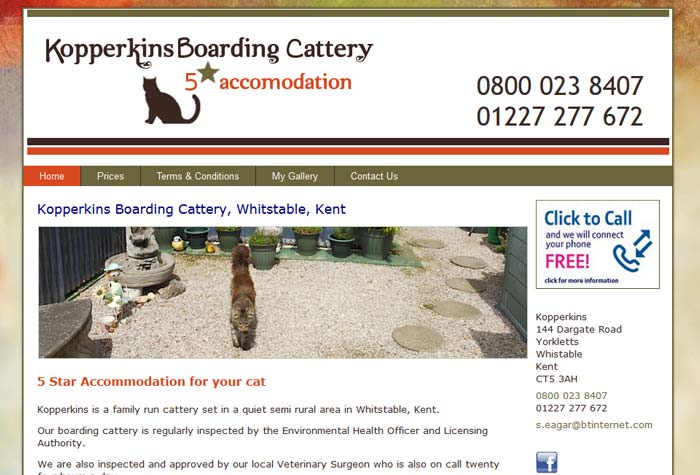Screenshot of the "Copper Kittens Board and Cattery" Website

- The website prominently features the title "Copper Kittens Board and Cattery," highlighting its five-star accommodation for cats.
- Two contact numbers are provided: 0800 023807 and 01227 277672.
- The website's color scheme predominantly uses shades of brown and red.
- The navigation menu includes sections such as Home, Prices, Terms and Conditions, My Gallery, and Contact Us.
- The cattery is located in Whitsnell, Kent, and is described as a family-run business set in a quiet, semi-rural area in the White Staple Camp.
- A detailed image showcases a tranquil garden area with rocks and a serene backdrop, featuring a cat.
- The facility is regularly inspected by a veteran surgeon, who is available on call 24/7 to ensure optimal care for the cats.